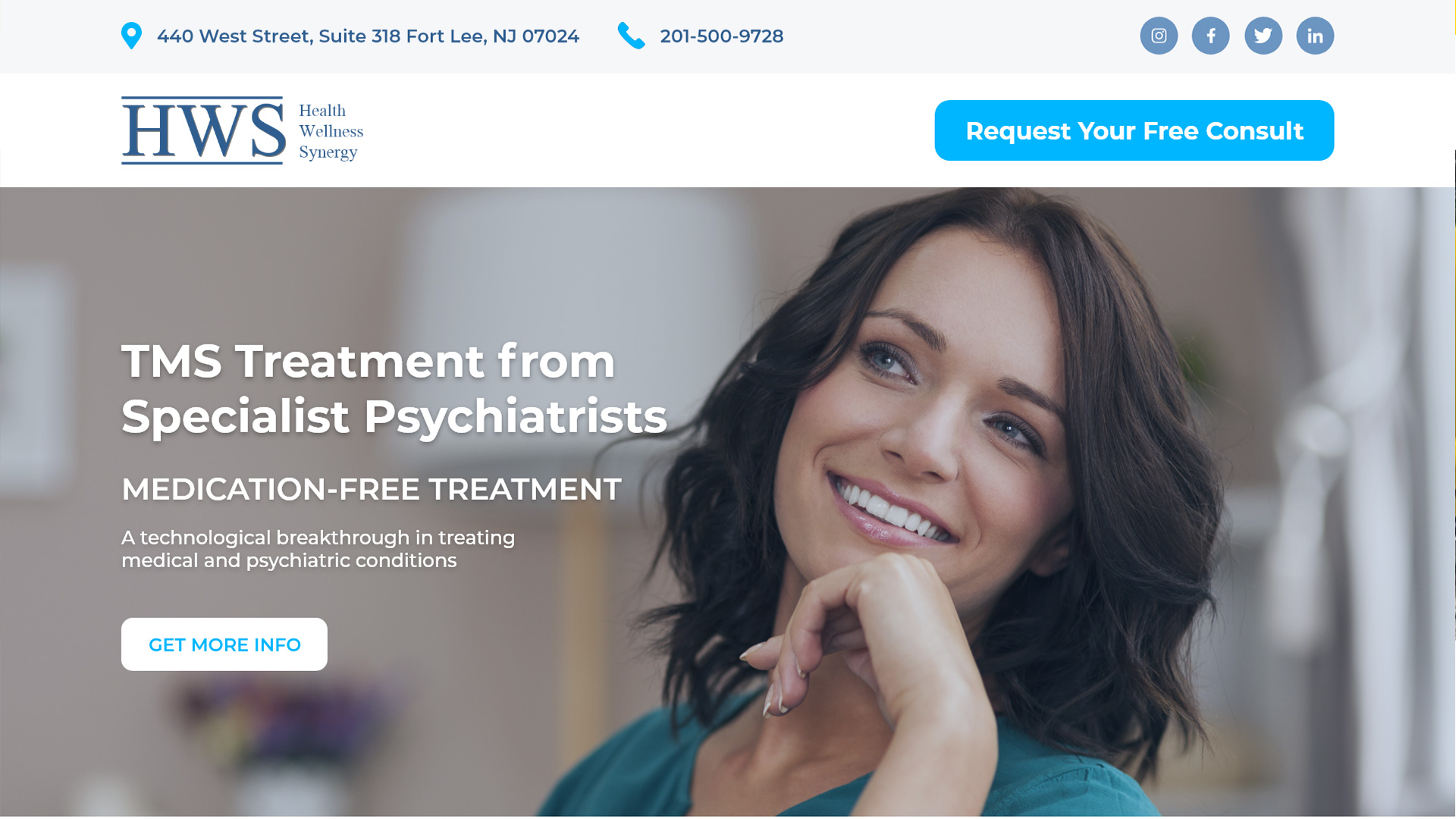**Blue Paz Health and Wellness Center**

**Address:** 440 West St, Suite 318, Fort Lee, New Jersey, 07024  
**Contact:** Phone: 201-500-9728  
**Social Media:** Instagram, Facebook, Twitter, LinkedIn.  
**Specializations:** Health, Wellness, Synergy

---

**Request Your Free Consultation Today!**

---

*Image Description:* A woman with short, shoulder-length hair smiles warmly at the camera, her left hand resting thoughtfully under her chin. Her gray eyes are striking, and she has a small mole under her left eye. She is wearing a green shirt and has pink lips, adding to her friendly appearance. Her nails are painted, enhancing her neat look. She appears to be sitting in a cozy room.

*Caption Text:* "TMS Treatment from Specialist Psychiatrist. Medication-Free Treatment and Technological Breakthrough in Medical and Psychiatric Conditions."

*Note:* The image was previously blurry, but it now clearly depicts the subject.